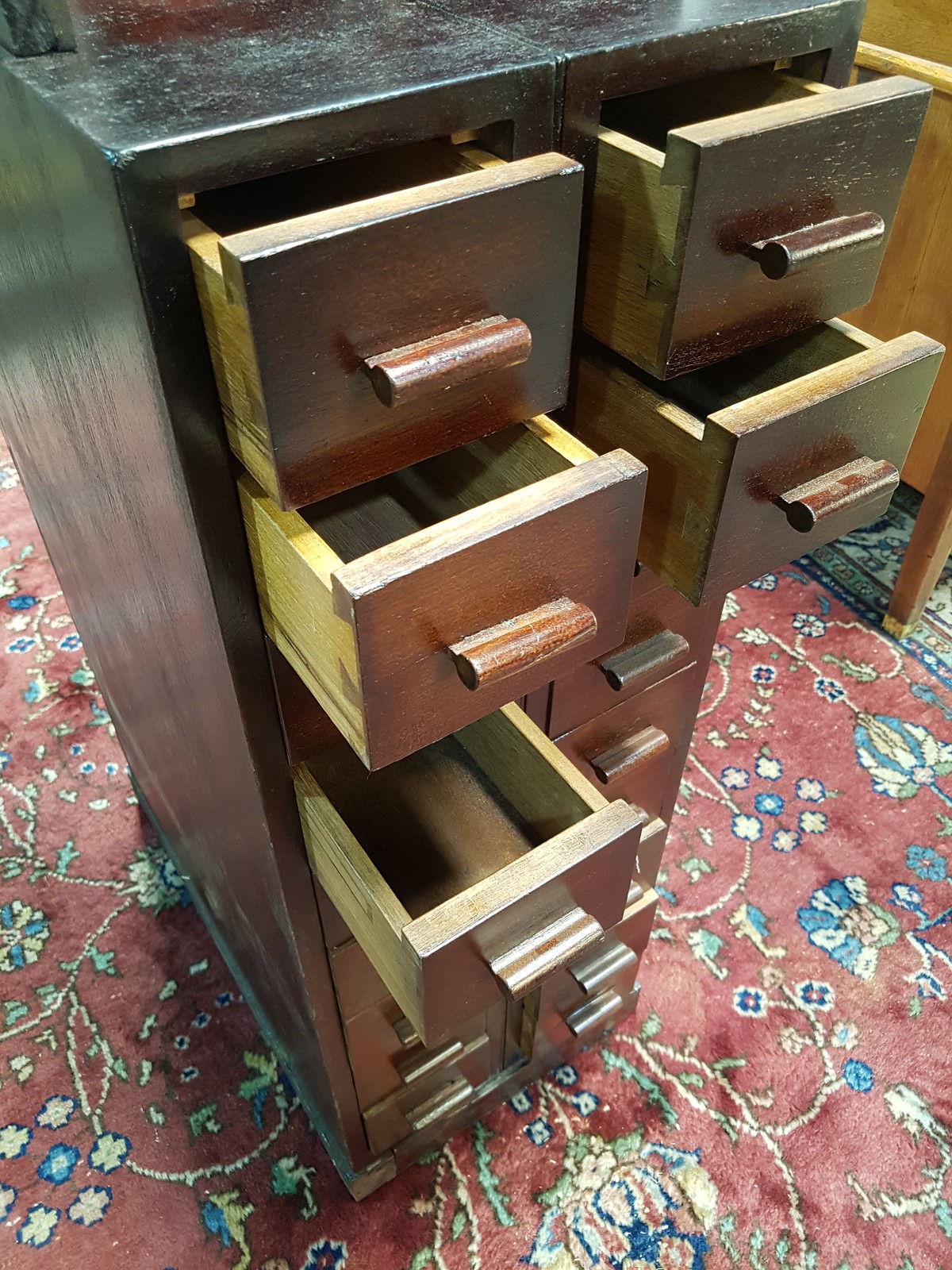This image captures a dark wooden, narrow, tall dresser with eight pairs of small drawers, arranged in two vertical rows. Each drawer features a long cylindrical handle extending horizontally. The drawers vary in their states, with the top four slightly ajar, none of them open to the same length. Additionally, one drawer on the left in the fourth row is noticeably more open. The piece of furniture stands on an ornate red carpet, adorned with blue and white flowers interwoven with green leaves, which gives it an oriental appearance. In the top right corner of the image, a brown shelf or cabinet is partially visible.